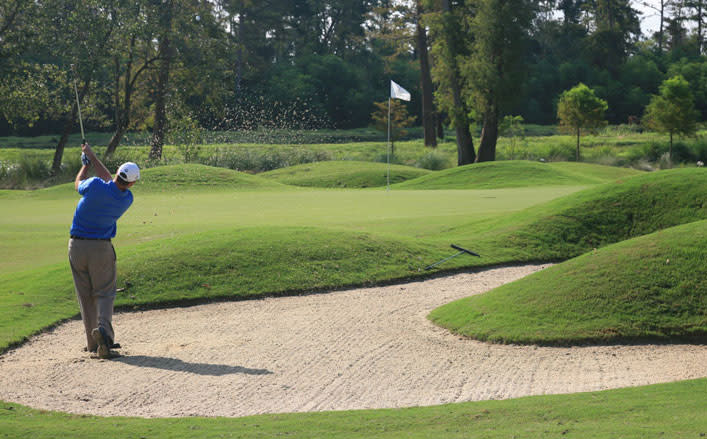A man is captured mid-swing while playing golf, showcasing his determined focus and precise mechanics. He wears grey pants, a blue top, and a white cap, and has a grey golf club in both hands. The image details the moment of impact as sand from the bunker is suspended in mid-air, highlighting the force of his swing. The golfer is positioned within a sand trap filled with grey sand, surrounded by lush green grass and gently sloping mounds. His target is the hole marked by a grey pole with a white flag in the center of a lighter green flat area. To the left, three tall green trees stand, with three more towards the center and two smaller trees on the right. Behind the flagstick, more mounded grass contours the landscape. The background features another expanse of grassy terrain leading into a dense green forest that stretches horizontally across the scene. Above, a grey sky casts a diffuse light over the course, suggesting a partially cloudy day.